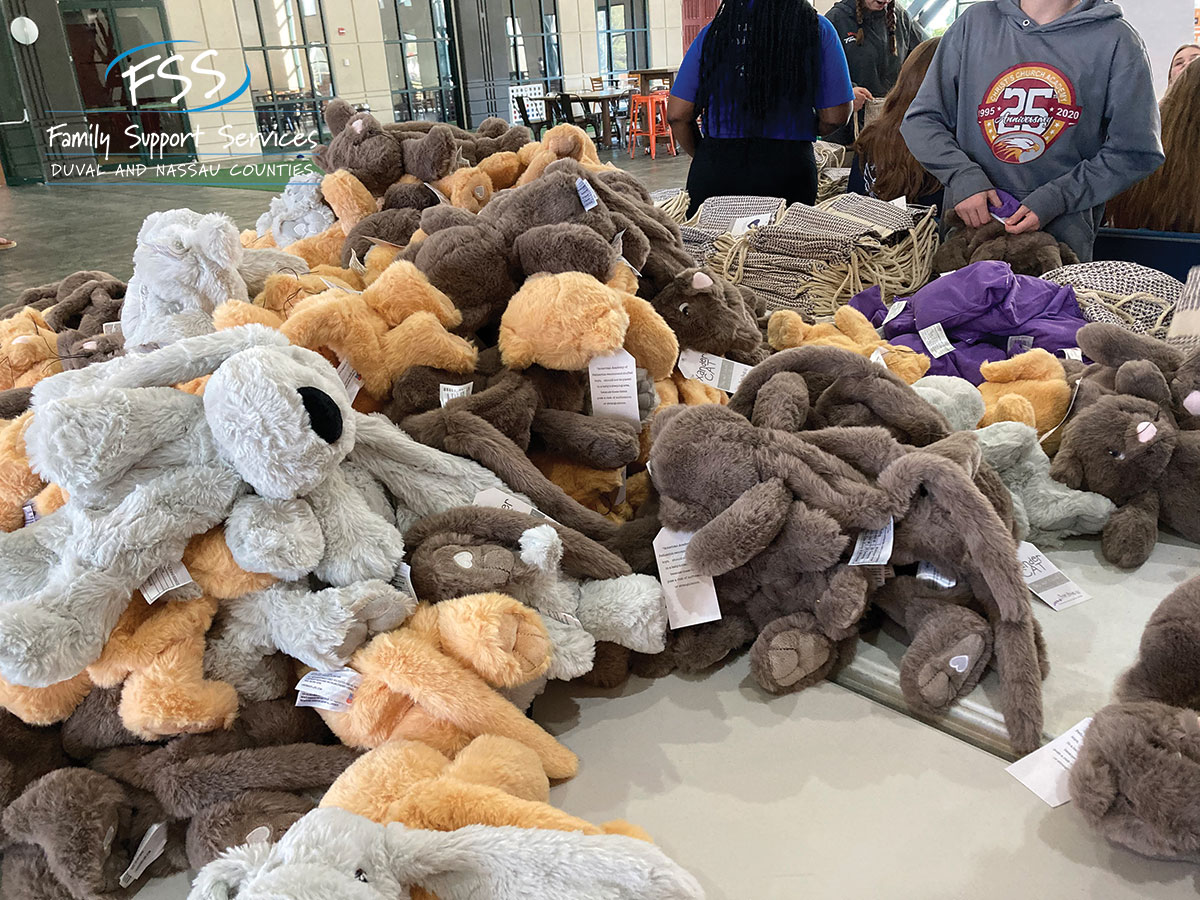The photograph, taken indoors, prominently features a large pile of assorted plush toys centrally placed on a series of foldable tables. The plush toys include gray and tan stuffed dogs, light to dark brown teddy bears, and possibly some plush monkeys, totaling dozens of items. Behind the plush toy display, in the upper right, a group of five to six people is partially visible, with some wearing sweatshirts and blue shirts. In the left background, additional tables, chairs, windows, and doors leading to another room are discernible. The photo also contains text on the left side that reads "FSS Family Support Services Duval and Nassau Counties." The scene resembles a charity event, likely aimed at supporting children and families in need.